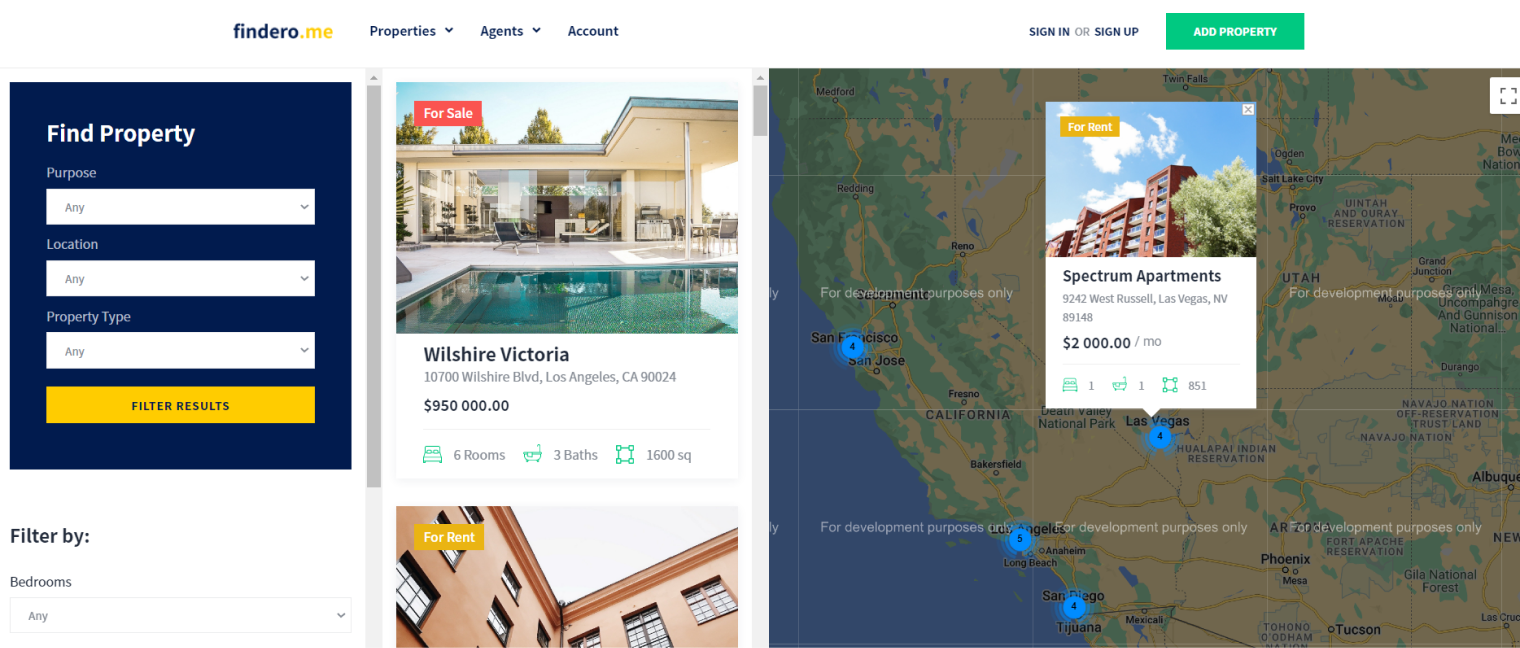The image depicts a website or app interface, structured in a widescreen format approximately two and a half to three times as wide as it is tall.

At the very top, there's a title area featuring dark blue text that reads "FindArrow and Dot Me," with the "Dot Me" portion highlighted in a suggested yellow. Following the title, there are three menu options in the same dark blue text: "Properties" with a down arrow, "Agents" with a down arrow, and "Account."

On the far right, additional options are presented: "Sign in" or "Sign up" in bold dark blue text. Adjacent to these options is a medium green horizontal rectangle button with white text that reads "Add Property."

The main area of the interface is divided into three sections. The first two sections occupy the left half of the screen:

1. **Find Property**: This section allows users to input details such as purpose, location, and property type. It also includes a filter option and a button labeled "Filter Results" at the bottom.
2. **Listing Options**: Positioned in the center, this section appears to display the search results or listings based on the criteria entered in the "Find Property" section.

The right half of the screen is dedicated to a map filled with bright blue pins. This particular map focuses on California, displaying four property options along the West Coast.